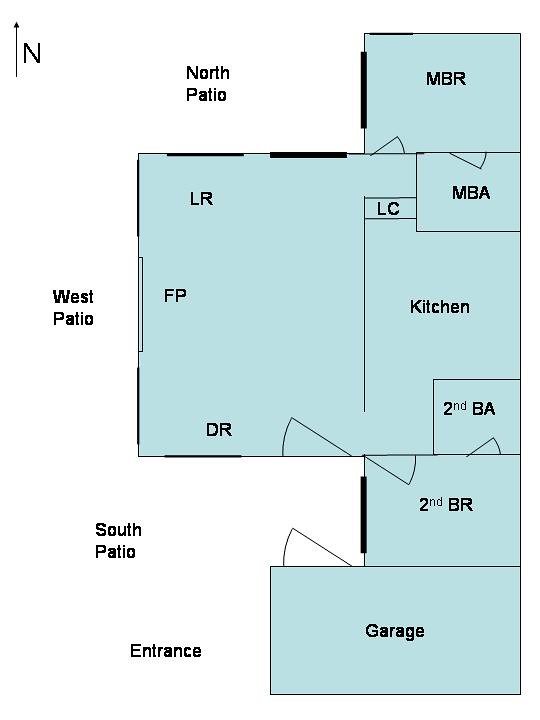This detailed floor plan features a highly organized layout with clear demarcations in black lines for each room and consistent blue fill with black lettering. The north side of the plan is indicated with a black arrow labeled "North Patio," which includes the Master Bedroom (MBR). 

Adjacent to the MBR, you'll find the Master Bathroom (MBA) and a large closet (LC). The central area of the plan includes a spacious kitchen and a cozy living room equipped with a fireplace, seamlessly connected to a dining room. 

On the west side, there's a second bathroom conveniently located for guest use. The south patio offers access to a slightly smaller second bedroom. Additionally, the entrance to the building is through a sizable garage positioned at the far end of the layout.

Overall, the floor plan illustrates a well-thought-out space featuring two bedrooms and two bathrooms.